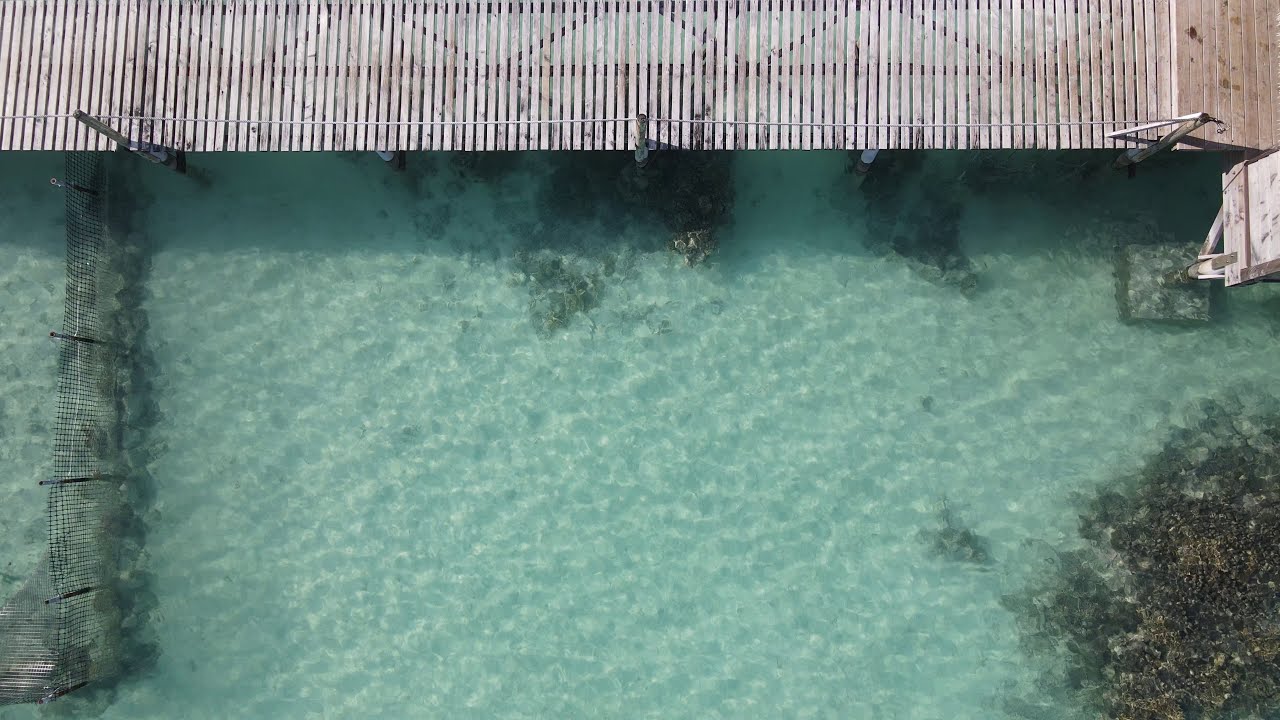This aerial view captures a tranquil waterscape, dominated by a slightly green-tinted water body that fills the majority of the image. Extending horizontally across the very top of the photograph is a wooden boardwalk or pier, constructed from brown wooden logs. The right end of the boardwalk appears denser and thicker, allowing glimpses of the water beneath it. To the left side of the water body, a metallic fence with netting extends vertically and submerges partially in the water. In the bottom right corner of the image, dark-colored moss or water plants are visible, adding a natural touch to the scene. The overall composition is devoid of people, highlighting the serene and undisturbed nature of the setting.